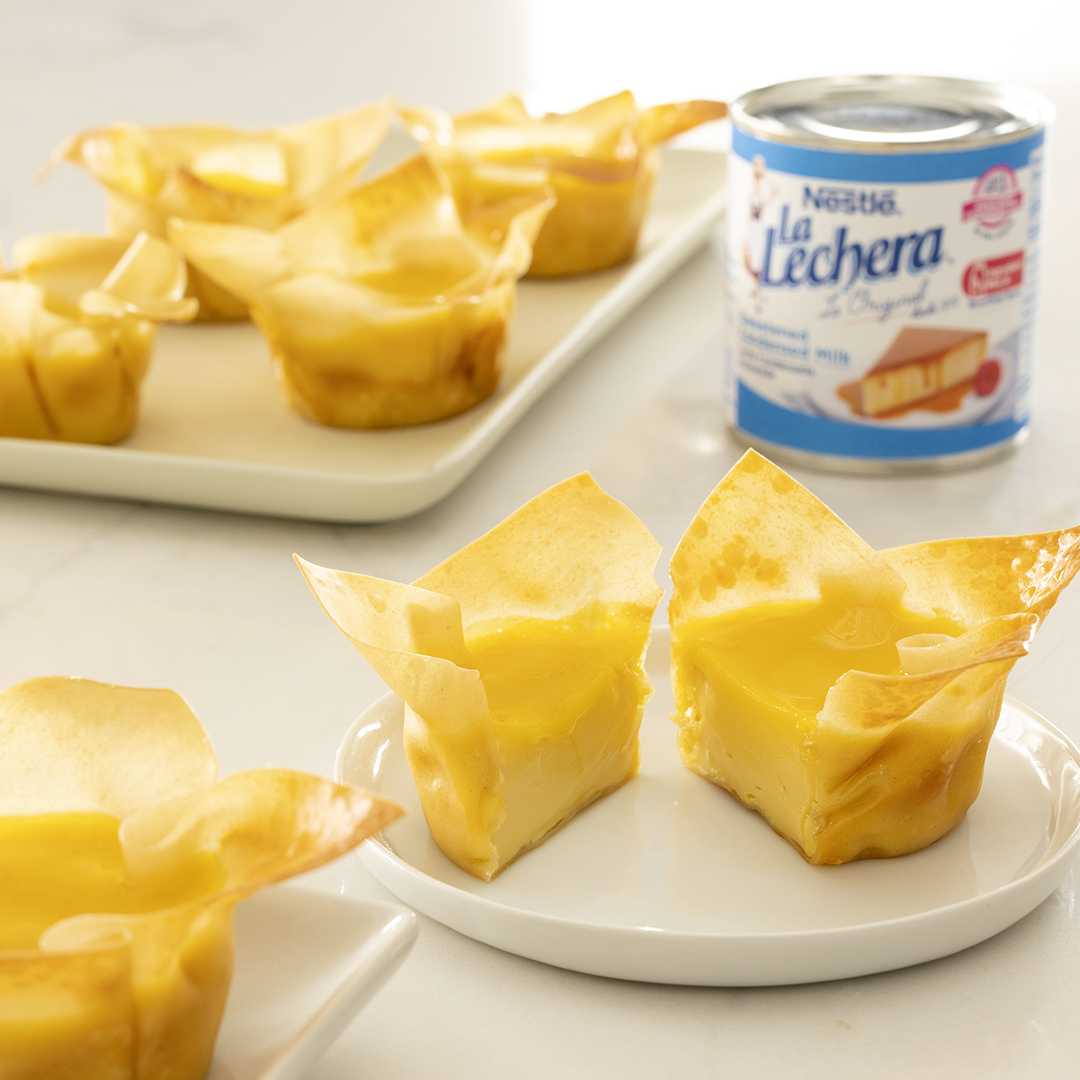This photograph showcases a delectable assortment of mini cheesecakes crafted with Nestle La Lechera sweetened condensed milk. The scene is set on a pristine white table, giving the image a clean, inviting look. At the forefront, a circular plate prominently features a mini cheesecake cut in half, revealing its creamy custard-like interior. The pastry shells, resembling phyllo or wonton wrappers, are golden brown and crispy, enveloping the rich filling. A smaller square plate at the bottom left corner also holds one of these enticing pastries.

In the background, a larger rectangular tray displays four more of these mini cheesecakes, all arranged in a visually appealing manner. To the upper right, slightly blurred to emphasize the foreground desserts, is a can of Nestle La Lechera. The can is white with light blue borders at the top and bottom, adorned with blue lettering and an image of a similar dessert, possibly flan, indicating its use as an ingredient. The entire composition suggests an advertisement or recipe thumbnail, perfectly capturing the mouth-watering allure of these mini cheesecakes.